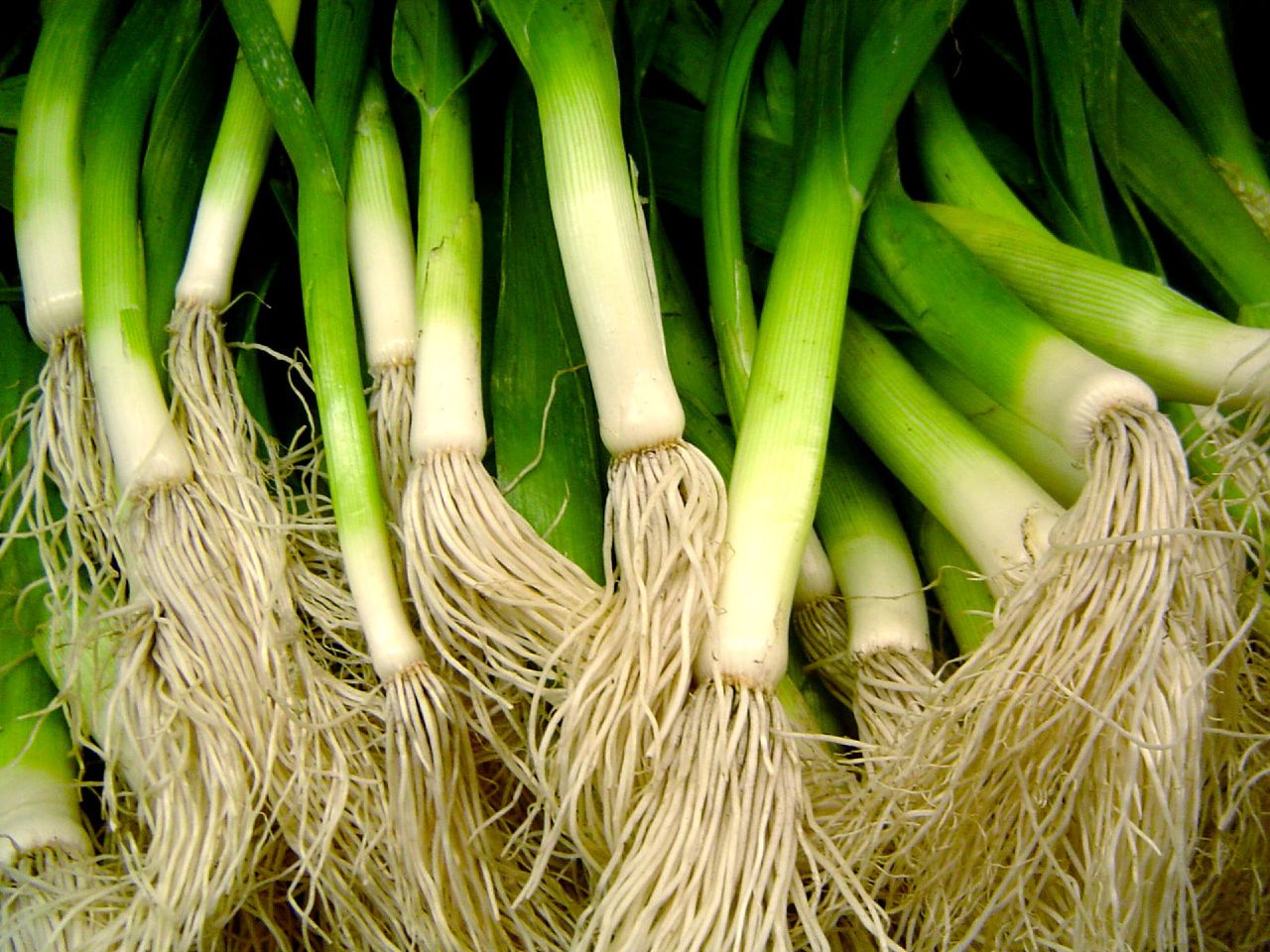This image is a close-up photograph depicting at least 22 green onions, also known as scallions, that belong to the lily family. The green onions are piled together with their roots facing downwards, cascading down the center two-thirds of the image and featuring visible dirt particles, suggesting they are unwashed. The white bulbous lower sections transition into the green, slender, vertical stalks. The composition of the image emphasizes the stringy, mop-like roots at the bottom, while the lush, green tops are clustered at the upper portion of the frame. The setting is ambiguous, possibly taken inside a grocery store, restaurant, or even a home kitchen.